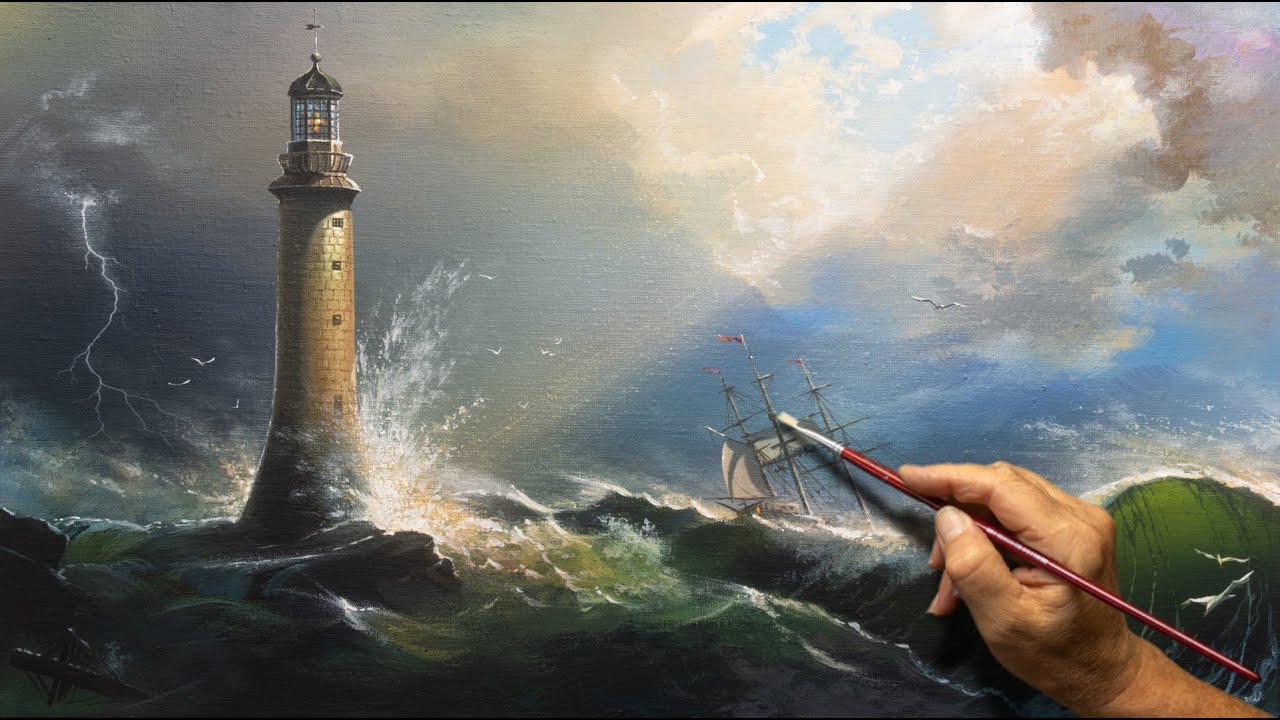The image depicts a very detailed and turbulent scene of an oil painting in progress, or at least staged to appear so. Central to the composition is a large, weathered lighthouse on a rocky outcrop, its once-white façade now a light brown, battered by the elements. Surrounding the lighthouse are massive, violent waves crashing against its base, colored in shades of green with white frothy crests. Above, a stormy gray-blue sky is electrified by a lightning strike, yet small rays of sunlight break through the clouds, illuminating part of the lighthouse. In the midst of this tempestuous sea, a white sailing ship struggles against the elements, seemingly caught in the chaos of the storm.

Notably, a clean, red-tipped paintbrush is visible near the bottom center of the image, held by a right hand that appears to be adding details to the canvas. The brush, conspicuously free of any paint, hints that the scene may have been crafted for a stock photo. The overall impression is that of a dramatic maritime scene, meticulously captured in the rough texture and rich colors typical of oil paint, with the artist's hand subtly reminding viewers of the ongoing artistic process.